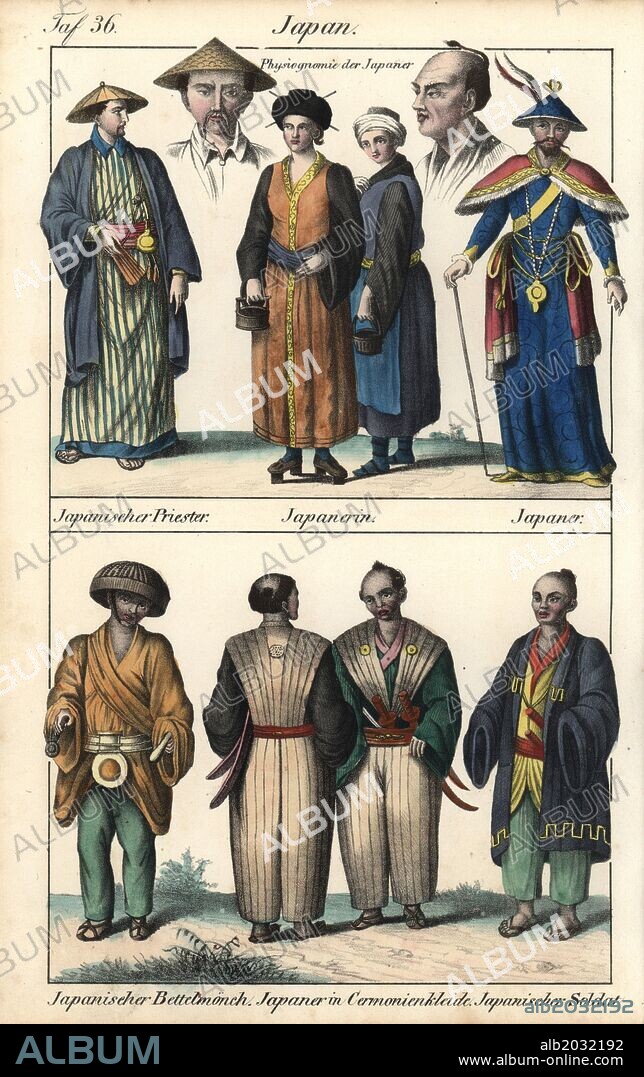The image is of the front cover of an album copyrighted by Album Online, with the URL www.album-online.com displayed at the bottom on a black border. The album cover is printed on off-white paper and prominently features the title "Japan" at the top in small black letters. The poster is divided into two sections: the top section depicts two Japanese subjects in traditional clothing, while the bottom section showcases eight standing Japanese men. Three of the men wear typical Japanese outfits with long flowing robes and pointy hats, and one is shown holding a weapon, suggesting a samurai depiction. Throughout the image, the word "ALBUM" is repeatedly overlaid in barely visible white letters, emphasizing the need for licensing.